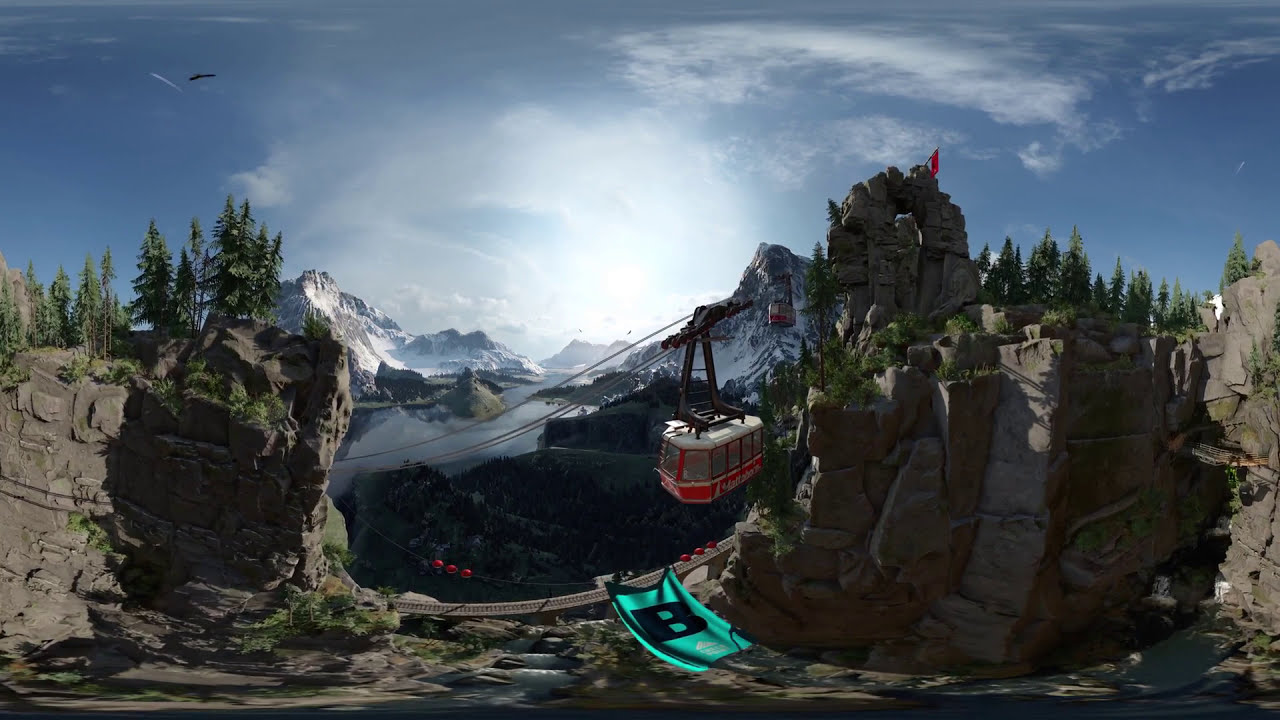The image is a highly detailed, likely computer-generated, scenic view featuring a bright blue sky with feathery white clouds. Dominating the background are tall, snow-capped mountain peaks, which add grandeur to the scene. Flanking the image on either side are sizable tan-colored cliffs with green grass and trees with brown trunks growing on them. 

In the foreground, there's a striking red and white cable car, attached to a black frame, traversing the sky on wires, giving a panoramic view of the landscape. Below this cable car, there's a turquoise or green ramp with a large, prominent letter B in dark blue or black. Additional black and white bobbers are visible further along the wires, contributing to the complex structure of the scene. 

Central to the image is a segmented arch formed by a mountain of rocks, allowing for pedestrian passage underneath. Beneath the arch, there's a distinctive drawbridge, sloping at its center, potentially serving as a railway bridge with visible train tracks. At the bottom, there's a water body surrounded by stones and greenery on both sides, harmonizing the natural and constructed elements of the scene.

To the right, a red flag flutters above one of the cliffs, providing a vibrant focal point. Intriguingly, on the far right side of the image, there's a whimsical addition of a unicorn, adding an element of fantasy. Smoke is seen rising near the mountain area, enhancing the dynamic atmosphere of the scene. 

Overall, the image merges realistic and fantastical elements, featuring intricate details like the red and white cable car, the green banner with a large letter B, and the picturesque natural landscape, all set under a clear blue sky.